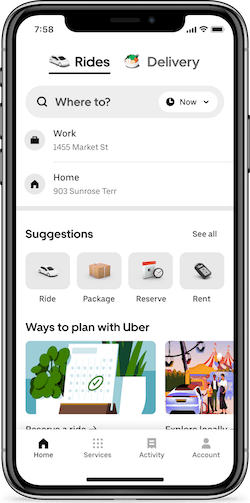The image is a detailed close-up of an iPhone's screen, prominently displaying the Uber app in focus. The time shown in the upper left-hand corner is 7:58. The layout is standard for an iPhone, with the main button positioned on the right-hand side and three additional buttons on the left. The Uber app interface is clearly visible, showing its primary sections: "Rides" and "Delivery" at the top. The "Rides" section is highlighted, identifiable by a white car icon, while "Delivery" features a symbol of food. At the top of the screen, a search bar labeled "Where To" invites the user to input a destination. 

Within this search bar, there is a drop-down menu titled "Now," suggesting the option to set a specific pickup time. The interface also displays pre-loaded addresses for "Work" and "Home," facilitating quick selection. Below these, there is a section titled "Suggestions," followed by another one labeled "Ways To Plan With Uber," offering users diverse planning and travel options. The overall image captures a user-ready moment within the Uber app, emphasizing its user-friendly design and functionality.